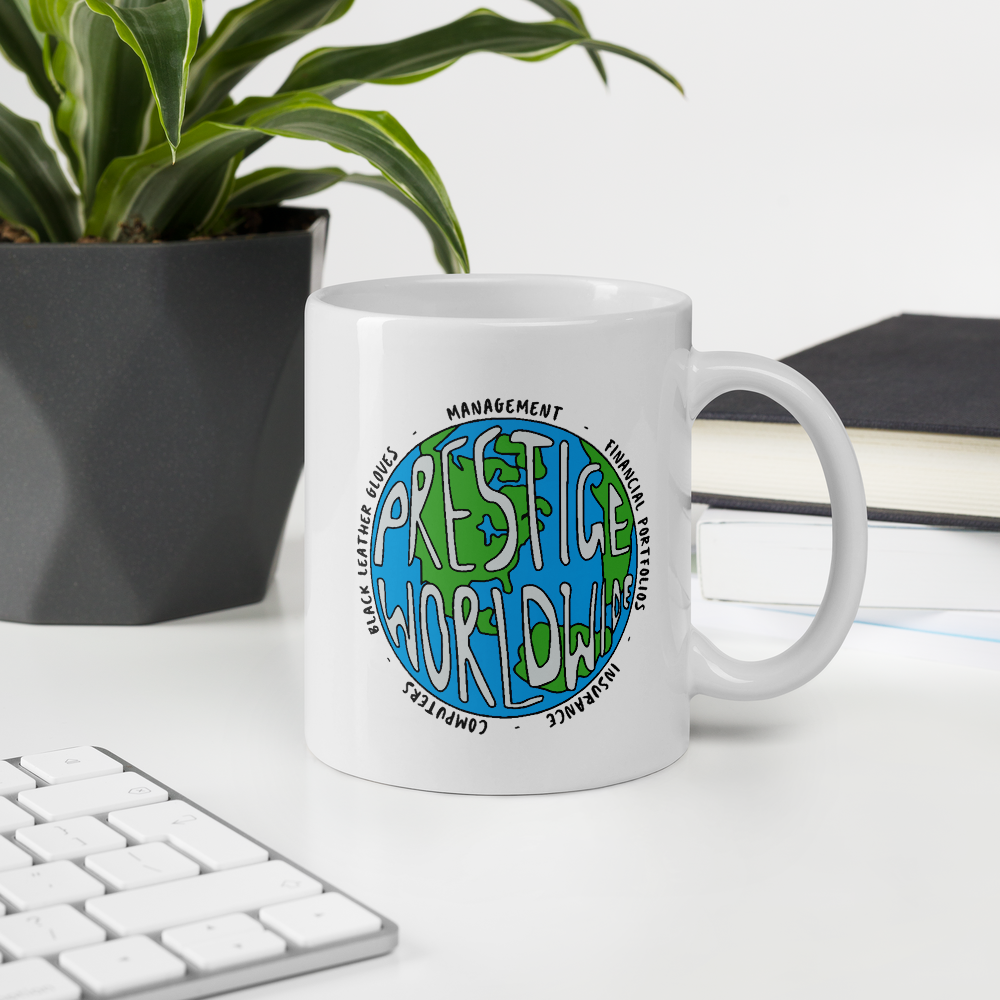In the center of a white table, there is a coffee cup prominently featuring a blue and green globe logo with white lettering that reads "Prestige Worldwide." This promotional cup showcases various business-related notes around the globe, including "management," "financial portfolios," "insurance," "computers," and "black leather gloves." Surrounding the coffee cup is a partial view of a separate, white-keyed keyboard. In the upper left side of the image sits a dark-colored pot with a green corn stalk plant, adding a touch of nature to the scene. A black book with no visible title is positioned in the background, contributing to the monochromatic theme of the photograph. The overall image is predominantly gray and white, with the vibrant coffee cup and green plant providing the main bursts of color.